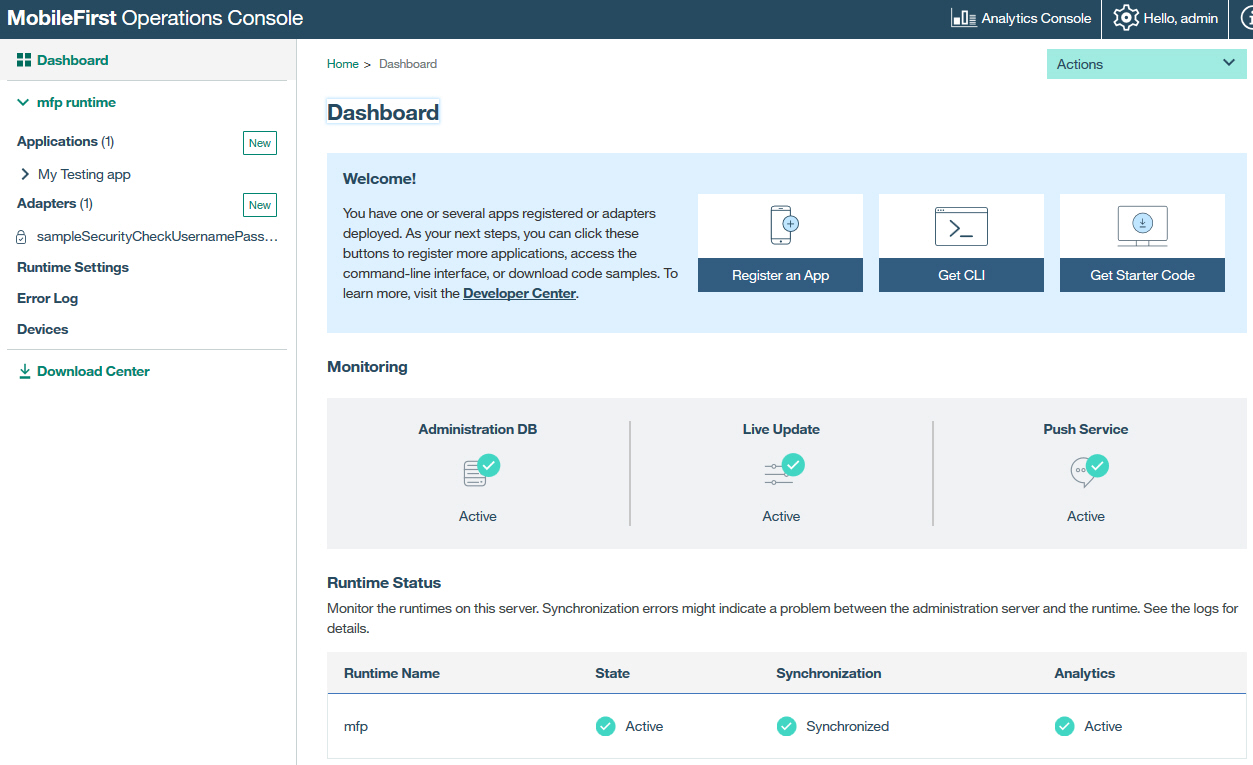A detailed screenshot of a computer monitor displays a user interface of the Mobile First Operations Console. The top of the screen features a dark green-gray bar. On the left side of this bar, bold white text reads "Mobile First Operations Console." On the right, the text "Analytics Console" accompanies a bar graph icon, followed by a vertical white line, a gear icon, and the words "Hello Admin" in white. 

Below this bar, a turquoise colored drop-down box labeled "Actions" in black text stands out. Along the left side, a vertical white column hosts several labels: "Dashboard," "MFP Runtime," "Applications (1)," with an adjacent "New" button. A right arrow points to "My Testing App" under the Applications section.

Next, the section labeled "Adapters" shows one adapter and another "New" icon to the right of it. Beneath this, a padlock icon accompanies the text "Sample Security Check (Username Pass)." Further down, bold labels include "Runtime Settings," "Error Log," and "Devices," followed by a "Download Center" icon in blue-green with a download arrow on the left.

The main center section on a white background prominently displays "Dashboard" in bold black lettering. A light blue rectangular banner runs across this section, greeting the user with a bolded "Welcome." It informs the user they have several apps registered or adapters deployed. To the right, options include "Register an App" with a phone icon, "Get CLI" with a file folder or computer monitor icon, and "Get Starter Code," which features a computer monitor icon with a blue download circle.

Under this banner, the bold word "Monitoring" appears on the left side, next to a horizontal light gray bar. In bold black text, the labels "Administrative DB," "Live Update," and "Push Service" are situated across the center, each marked by a gray icon featuring a green circle and a white checkmark in the upper right corner. At the bottom, the words "Active" appear in black for each section.

The final label, "Runtime Status," present in a gray bar, lists columns such as "Runtime Name," "State," "Synchronization," and "Analytics." Below, entries like "MFP Active," "Synchronized," and "Active," are each accompanied by a green dot with a white checkmark.